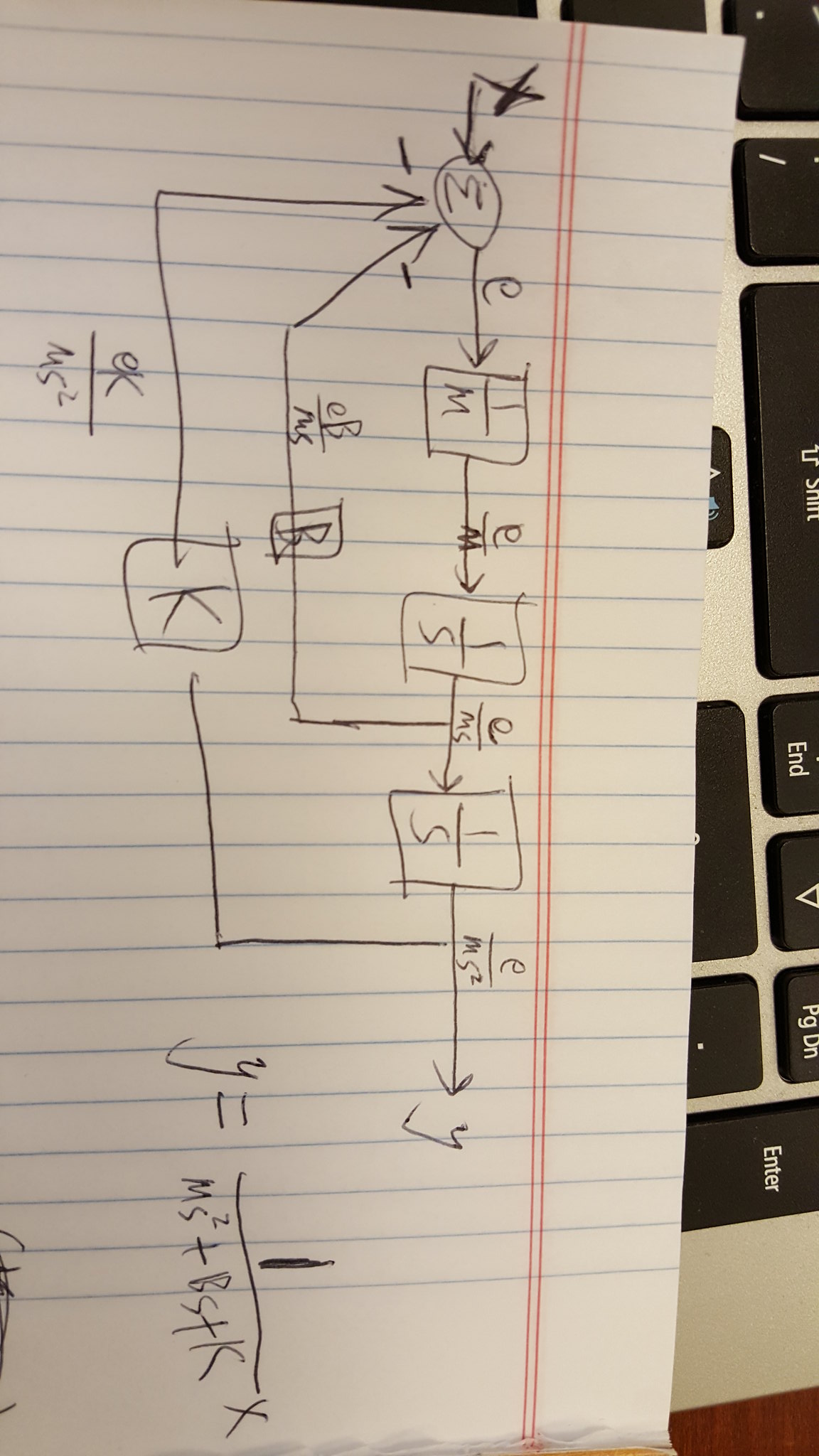Indoor photograph turned 90 degrees clockwise showing a detailed technical diagram on a notebook page occupying the center and right side of the image. The diagram consists of a series of interconnected elements and equations drawn diagonally across the page. Starting from the top-left corner (now the bottom-left due to the rotation), there is a circular symbol integrated into an equation, followed by a downward line connecting to a rectangle containing the fraction 1/M. Another line extends from this rectangle to an adjacent rectangle labeled 1/S, and yet another line links this to a second 1/S rectangle. From here, a final line points down to a symbol marked with Y.

Beneath this sequence, there is an annotated left margin. At the bottom center, we see a rectangle with the letter B, flanked by vertical lines running through it, which then diagonally connect back to the initial M or E symbol at the start of the equation. An additional line intersects between the two 1/S fractions, with an equation E/MS written above it.

To the far left, another rectangle labeled K is positioned with a vertical line descending about an inch before making a right-angle turn to join with the lines of the primary diagram. Additionally, on the right edge of the photograph, a section of a keyboard is visible, featuring black keys set against a silver background. No other text or print is discernible in the photograph.